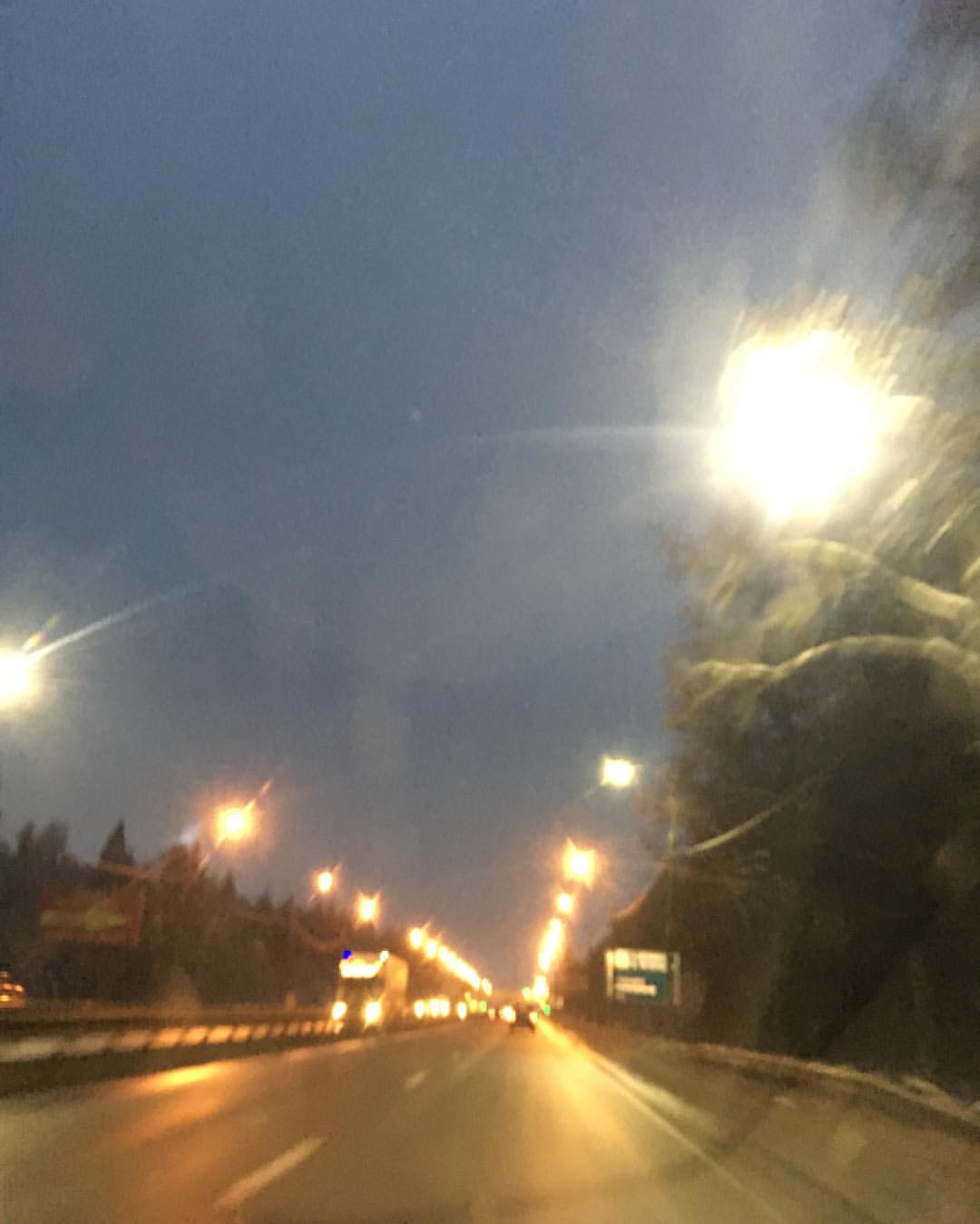This color photograph captures a highly blurred, nighttime scene of a wide highway or street in an urban area. The sky, dark blue and enveloping about 80% of the composition, suggests that the image was taken either at night or just after sunset. The blur, possibly caused by the photo being shot through the window or windshield of a moving vehicle, adds an abstract, dynamic quality, making fine details difficult to discern. Streetlights line both sides of the road, their reflections gleaming off the pavement and broken white lines marking the lanes, creating a sense of depth and perspective.

On the right side of the image, a very large, blown-out streetlight occupies the upper corner, emitting rays that scatter across the scene. Below it, there's an area clustered with trees. To the left, a row of buildings peeks out from behind some shrubbery, while a potential walkway or path is faintly visible. Further along the left shoulder, a reddish billboard stands near the barrier. The highway itself has at least three lanes, with vehicles, likely including a truck or bus in the closest left lane, heading towards the viewer with their headlights on.

There are also signs suggesting exit routes, one notably dark and possibly green with white lighting towards the center-right of the frame. The overall impression is that of a busy urban roadway, lit by artificial lights and bustling with evening traffic, yet rendered almost dreamlike by the motion blur and reflection artifacts.